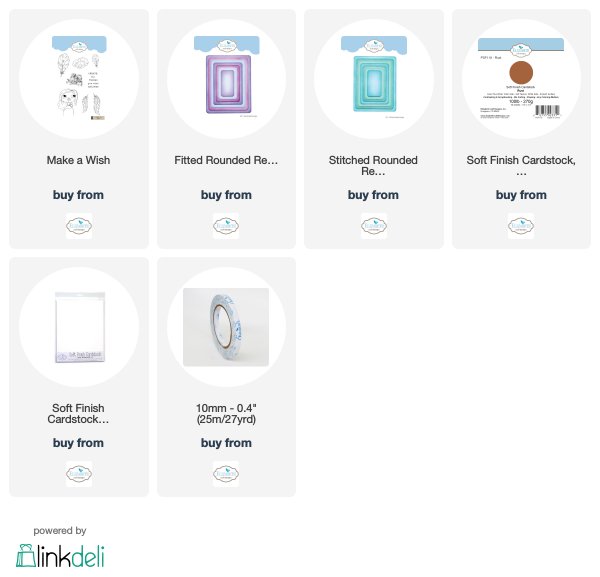The image depicts a section of a computer website featuring six distinct boxes set against a gray background. Each box contains an image and various pieces of text. 

1. The first box showcases an image of what appears to be a doll with accessories inside a white circle. The text adjacent to the image reads "Make a Wish" and "Buy from," though the specific retailer cannot be read due to the small size of the text. At the bottom, it includes an icon of a shopping bag and a "Powered by Link Deli" label.

2. The second box has a rounded frame with the letters "RE" displayed in purple. It includes the text "Buy from."

3. The third box is similar to the second, but the frame is green and labeled "Stitched Rounded." It also includes "Buy from" text.

4. The fourth box presents an image labeled "Soft Finish Cardstock" with a small brown dot inside a white circle. It has numerous small writings along with an SKU number, though the text is difficult to read due to its size.

5. The fifth box is another "Soft Finish Cardstock" labeled image, but this one has a purple notepad in the design. It includes "Buy from" text.

6. The sixth and final box displays a blue ring with the dimensions "10 millimeters 0.4 inches" accompanied by "Buy from" instructions. Like the first box, it also mentions "Powered by Link Deli."

Overall, this website section seems to offer various items for sale, each accompanied by purchase instructions and visually distinctive elements to differentiate the products.